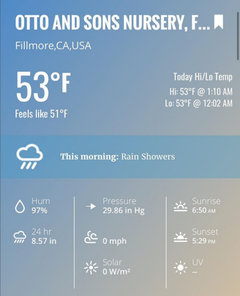This image is a detailed weather indicator screenshot for Oto and Sons Nursery in Fillmore, California, USA. At the top, bold white text displays the name "OTO AND SONS NURSERY F..", followed by a bookmark icon. Below this, location information "FILLMORE, CA, USA" is shown in capital letters.

The current temperature is 53°F, with a "feels like" temperature of 51°F. Today's high and low temperatures are both noted as 53°F, with the high recorded at 1:10 AM and the low at 12:02 AM.

A key weather summary for the morning features a cloud icon with rain, accompanied by the text "Morning rain showers" in white, set against a light blue highlighted bar.

Further details are organized into three columns at the bottom:

1. **Humidity**: 97%
2. **Rainfall (24 hours)**: 8.5 inches
3. **Pressure**: Atmospheric pressure in unspecified units
4. **Wind**: Measured in miles per hour
5. **Sun**: Not specified

Additionally, on the far right, sunrise and sunset times are provided along with the UV index percentage.

This comprehensive weather snapshot offers a complete overview of the current and expected conditions at this specific location.